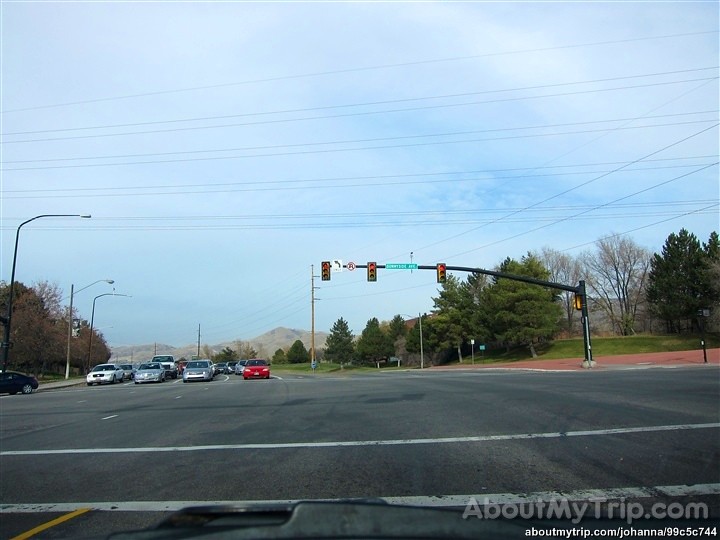A horizontal photograph captures the view from behind the wheel of a black car positioned at a stop sign, revealing the vehicle's hood and displaying text at the bottom right corner from "aboutmytrip.com," including a specific URL indicating a dash cam recording. The scene encompasses a clear day with a partly cloudy sky, set against a backdrop of pine trees and a barren mountain range in the distance. In the adjacent lanes, three stopped passenger cars—a white car and two silver cars—are visible on the left, with a red car situated in the turn lane. A black car can be seen making a right-hand turn from the far right lane.